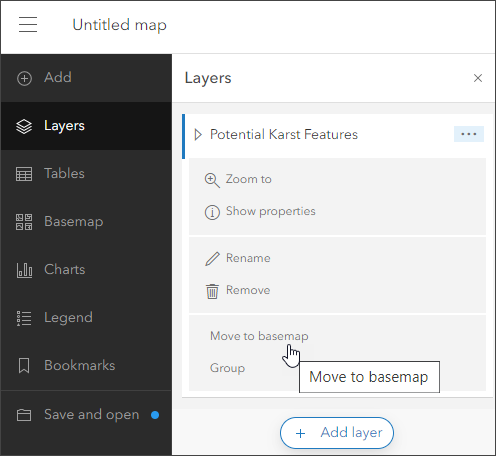Screenshot of a Mapping Application Interface

The image is a screenshot of a map-oriented application. At the top of the interface, a minimalist menu icon consisting of three horizontal lines is positioned on the left, followed by the title "Untitled Map" on the right, all set against a white background. Directly below this, a sidebar menu with a darker gray background and lighter gray text lists several categories: Add, Layers, Tables, Space Map, Charts, Legend, Bookmarks, and Save and Open. The "Layers" category is selected, evident by its highlighted darker black background. 

To the right of this sidebar, a main panel displays further details, featuring a light gray to white background. The title "Potential Karst Features" is prominently displayed, followed by options such as "Zoom to," "Show properties," "Rename," "Remove," "Move to base map," "Group," and a prominent button labeled "Add Layer" at the bottom. This panel appears designed to offer functionality specific to managing map layers within the application.